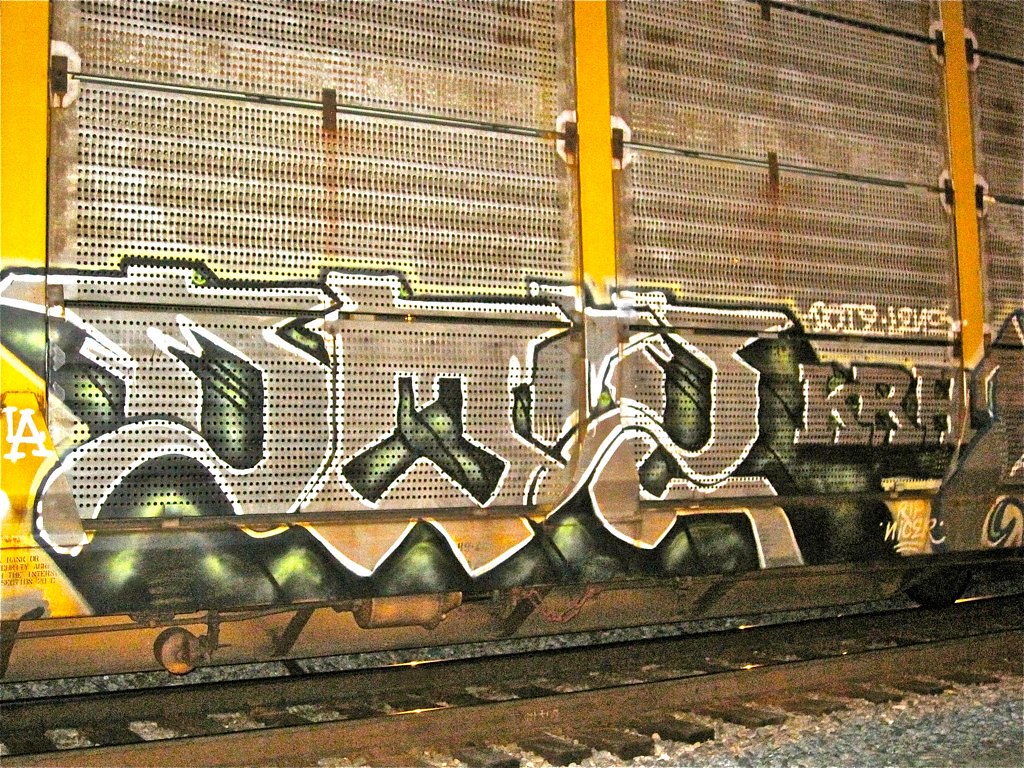The image depicts the side of a metal railway car with a gravel foreground leading up to the train tracks. The railway car, designed with a metal grate-like exterior, features distinct yellow vertical bars and rusted latches. The side of the car is adorned with graffiti; predominantly gray letters outlined in black with white highlights, set against a green painted background. To the left, there's a small white painting resembling the LA logo, akin to the Dodgers' symbol. In the central section, the larger graffiti letters are unidentifiable, but further to the right, clear block letters in the same gray color spell out "KRH." There's also mention of a smaller white inscription reading "RIP" and a drawing off to the side.